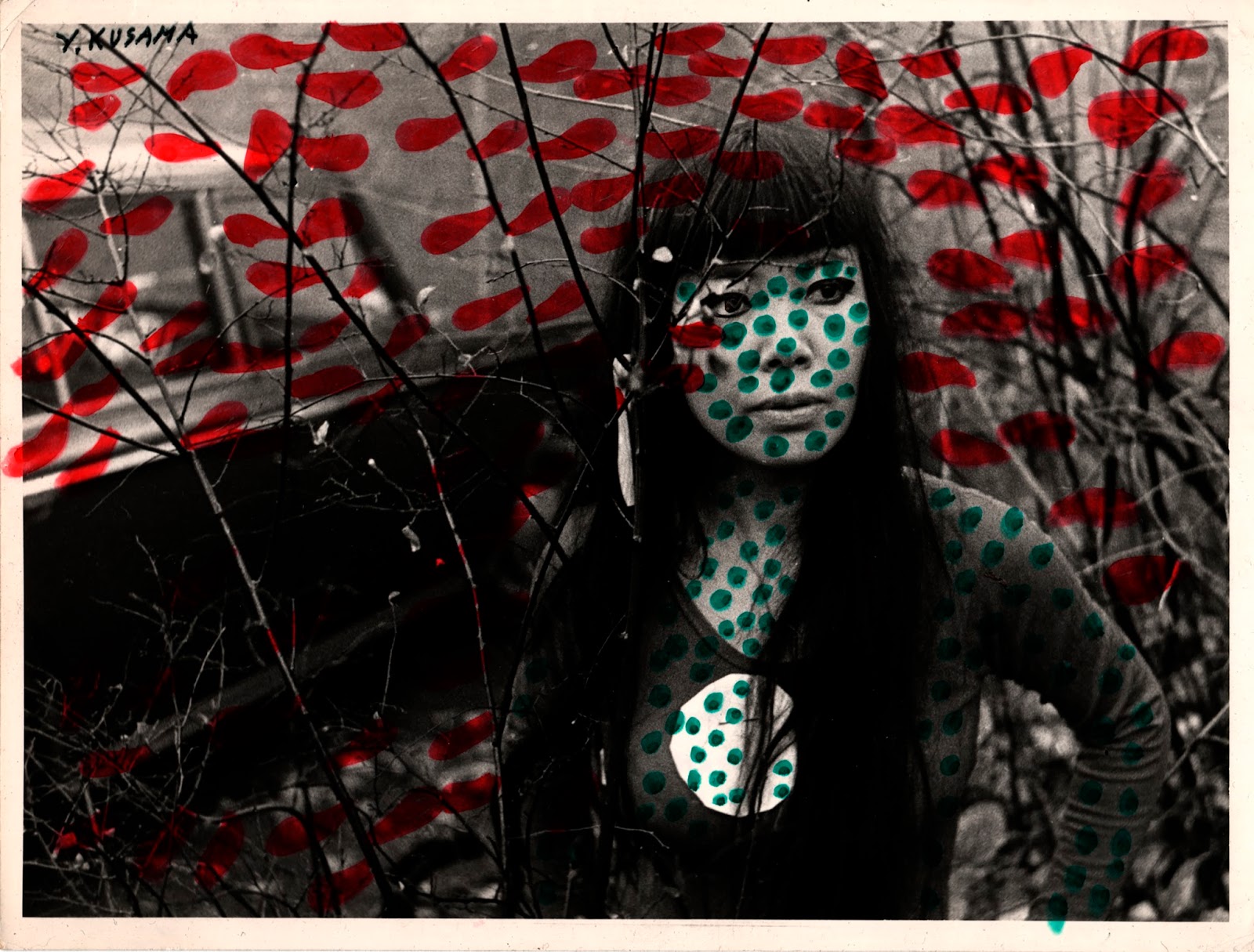The image is a photorealistic yet artistically altered black and white portrayal of an Asian woman captured from the waist up. She stands in front of predominantly bare branches or shrubbery, which have been painted with red oblong shapes, resembling leaves. The composition includes a muted, vintage-style car with a white top and black bottom to the left in the background. The woman, who has long, jet black hair with choppy bangs, heavy eyeliner, and thick eyebrows, gazes slightly off to the camera's right. She is adorned in a gray, skin-tight long-sleeved T-shirt under a black thin vest or dress, both of which are splattered with vibrant green dots of paint. Additionally, there's an ornamental piece hanging from her hair on the right side. The top of the painting is inscribed with the word "Yikusana" or "Yakushima," adding another layer of mystery to this eerie yet compelling piece.